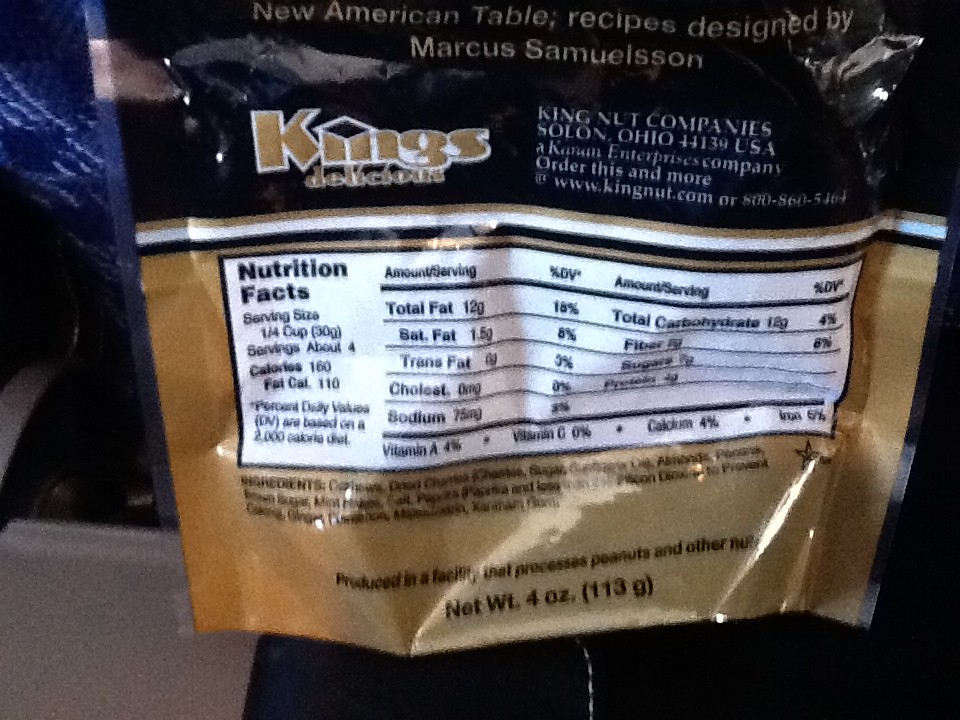This detailed photograph showcases the back of a snack container with a packaging design predominantly featuring black at the top and gold at the bottom. The package prominently displays "New American Table Recipes designed by Marcus Samuelson," and it is produced by King Nut Company, Solon, Ohio, 44139, USA, with the brand name "King's Delicious." The packaging includes both nutritional information and ingredients in black lettering, but some details are difficult to discern due to the image's blurriness and bag folds. It is specified that the product was produced in a facility that processes peanuts and other nuts. The nutrition facts indicate a serving size of 1/4 cup (30 grams), with about 4 servings per container, totaling 160 calories per serving (110 from fat), 12 grams of total fat, 1.5 grams of saturated fat, 0 grams of trans fat, 0 milligrams of cholesterol, 75 milligrams of sodium, 12 grams of total carbohydrates, and 4 grams of protein. The vitamins and minerals include 4% Vitamin A, 0% Vitamin C, 4% Calcium, and 6% Iron. The back cover of the package also features a website, order information, and a blurred contact number. The background of the photograph includes some kind of blue fabric at the top and grey fabric at the bottom.